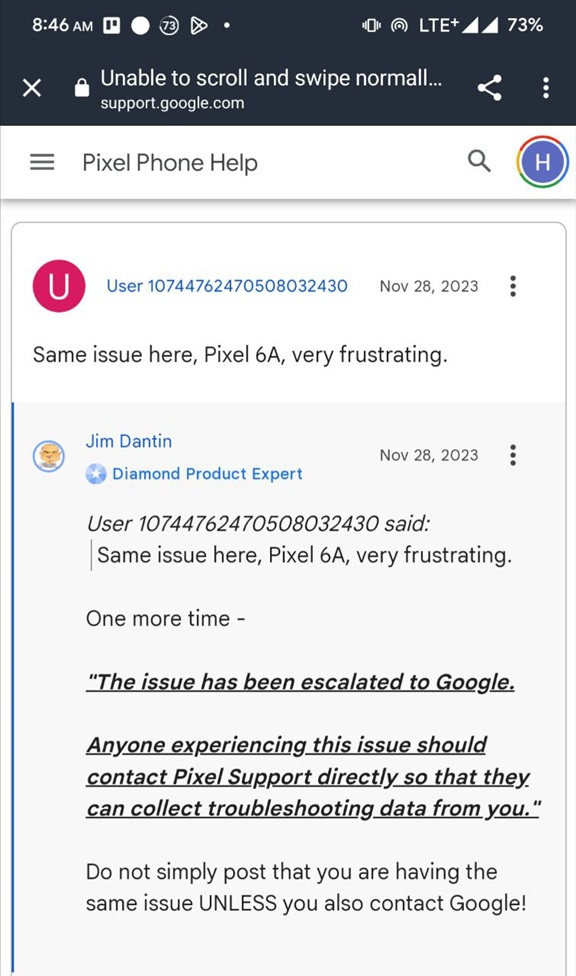Screenshot Description: A detailed view of support-related content on a Google Pixel phone.

The screenshot captures a Pixel phone screen where a user is navigating to the "Pixel Phone Help" category on the support.google.com website. The user is seeking assistance for an issue where the phone is unable to scroll and swipe normally. 

On the screen, an October 28th, 2023 comment from a user with the ID 10744762470508032430 is visible, stating, "Same issue here, Pixel 6a, very frustrating." In response, a Diamond Product Expert named Jim Danton replies on the same date, clarifying, "The issue has been escalated. Anyone experiencing this issue should contact Pixel support directly so that they can collect troubleshooting data from you. Do not simply post that you are having the same issue unless you also contact Google."

At the top of the screen, the status icons indicate the time as 8:46 AM, the device is in vibrate mode, has the Play Store app icon present, shows full LTE+ signal strength, and a battery level of 73%.

The user is attempting to find a solution for their malfunctioning swipe functionality and learning that contacting Google Pixel support directly is necessary to address this known issue.